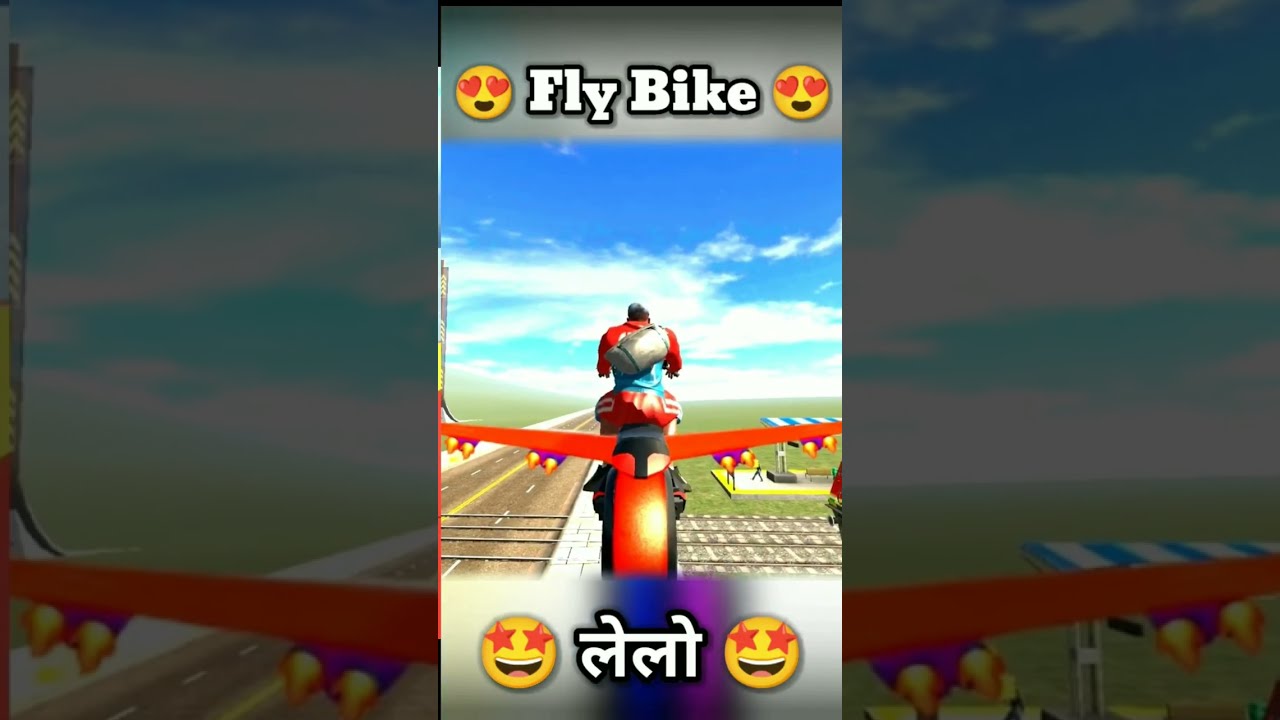The screenshot captures a vibrant, 3D scene from a video game, likely a mobile or possibly a console game due to its simplistic textures and geometry. The focal point is a character in an orange or red suit, complete with a brown duffel bag slung across their back, riding what appears to be a winged bike or a streamlined airplane with jet propulsions under its red wings. They soar over a landscape featuring intersecting train tracks and a divided highway, with expansive green fields stretching into the horizon under a clear blue sky dotted with white clouds. 

Framing the scene, the top of the image displays a gray bar with the bold white text "Fly Bike," each word capitalized and outlined in black. This title is flanked by yellow smiley emojis with heart eyes. Directly beneath this title is a word in Hindi, also accompanied by emojis, this time featuring happy faces with red star eyes. The bottom of the image also includes a similar gray bar. The combination of vivid imagery and playful elements creates an engaging and whimsical atmosphere, suggesting a lighthearted and adventurous game experience.